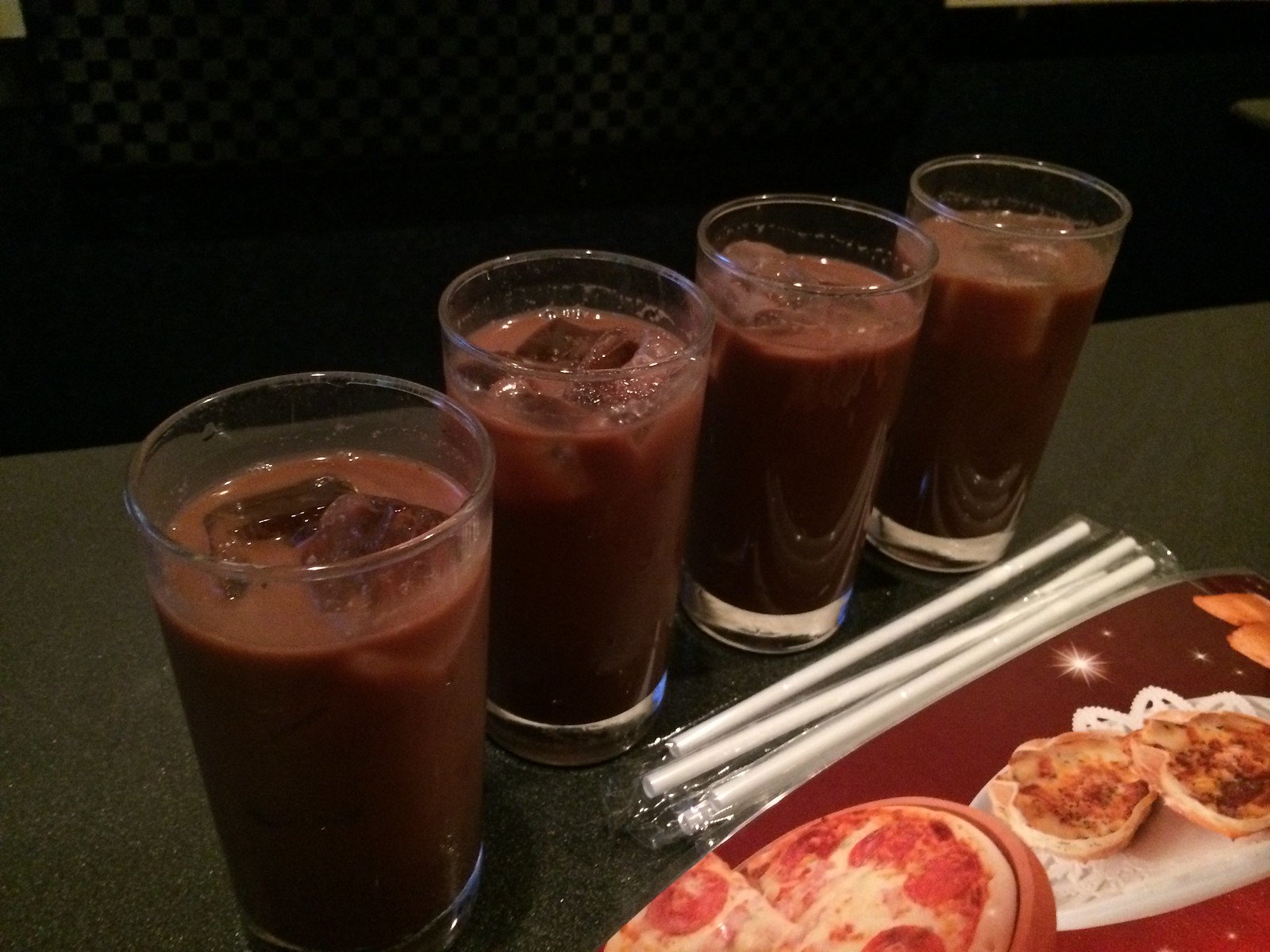The image depicts a restaurant table set for four, indicating a booth seating arrangement characterized by checkered backrests. Dominating the table are four identical glass cups, each filled about seven-eighths with a thick, dark brown drink that resembles a richly chocolatey soda or a deeply flavored milk beverage, possibly a unique variant like a Mexican chocolate drink. The glasses contain ice cubes and glint under the ambient light. Alongside, four straws remain in their wrappers, placed neatly next to the glasses. Centered on the table is a small pepperoni pizza resting on a tray, slightly tilted to one side. Further adding to the array of items are two hors d'oeuvres, described as brown pastry puffs, elegantly displayed atop a doily or plate. The lower part of the image exposes a fragment of a menu suggesting pizza options and possibly other items like quiches or mozzarella sticks. The overall composition and lighting suggest a casual dining experience, captured with a lot of color and no text.